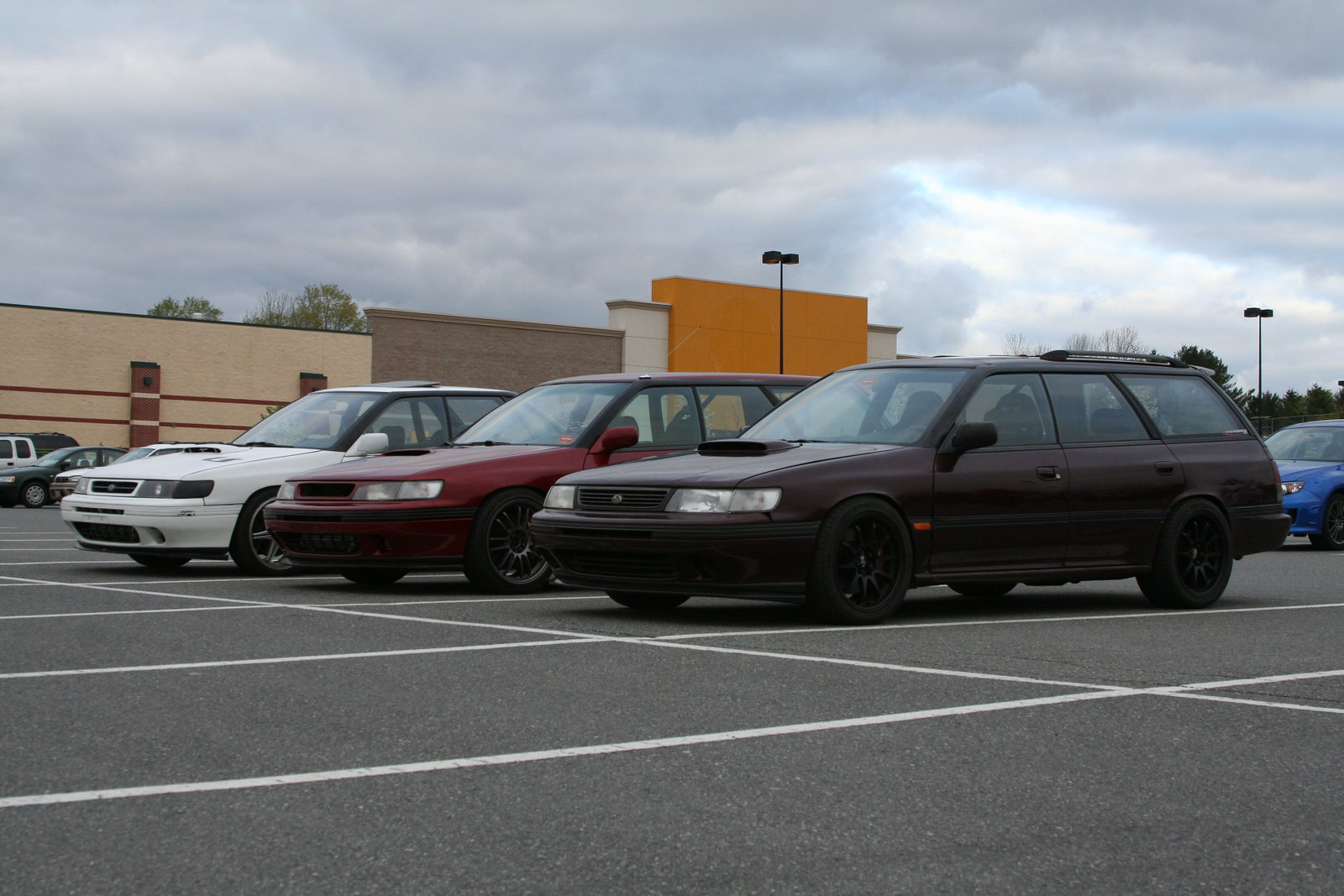In the image, which is taken during the daytime under an overcast, cloudy sky, a parking lot is seen in front of a complex building. The main building shows a combination of colors including orange, dark brick, creamy brown, beige, and pale red or burgundy lines or designs. The structure appears conjoined with walls of various colors: orange, white, beige, and brown. Behind the cars, there are some trees partially visible. In the foreground, there are three main SUVs parked in a row: the one on the left is white, the one in the center is a dark red or burgundy, and the one on the right is a deep maroon or chocolate color. Visible parking spaces are outlined in white stripes on black asphalt. Additionally, there are a few other vehicles in the next row: part of a blue car, a white van, and a black car. Two streetlamps can be seen near the building, one of which is illuminated. The overall scene suggests a calm, potentially rainy day ahead.